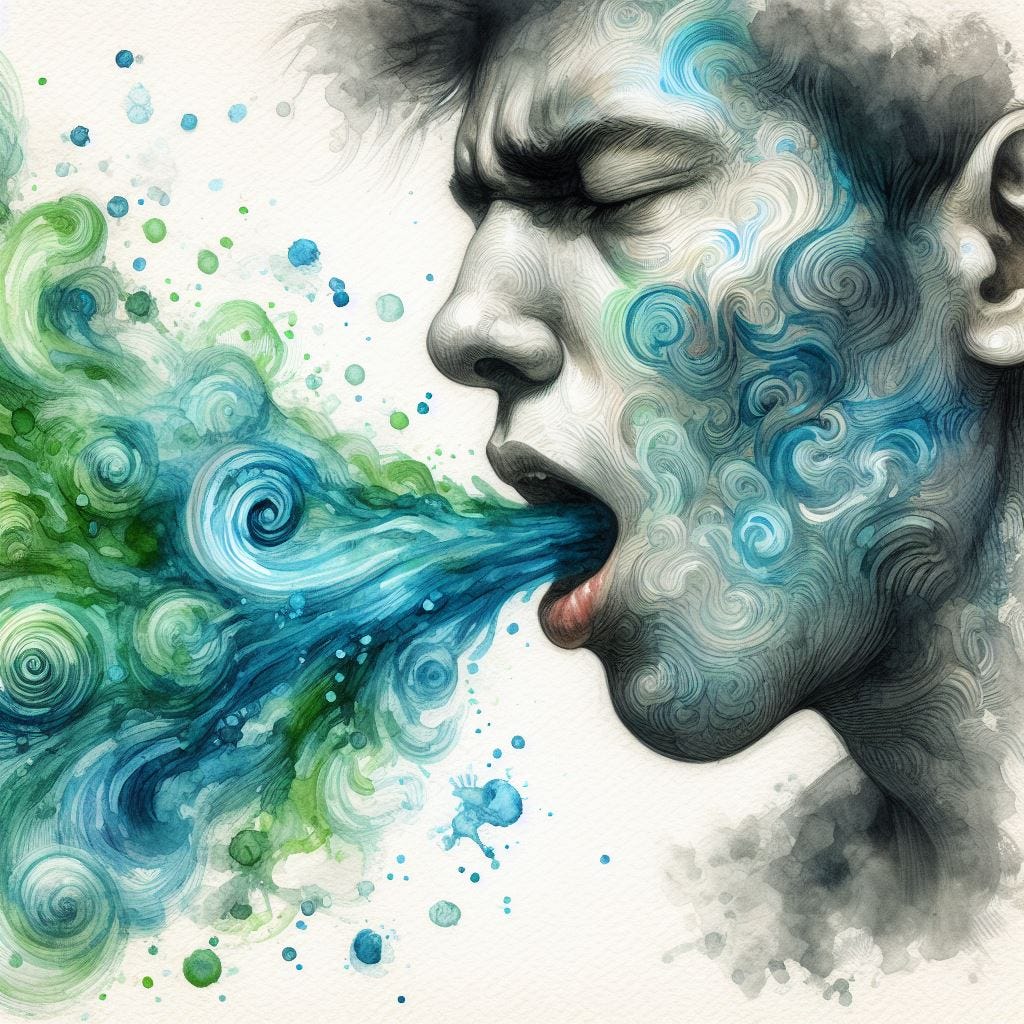The image is an abstract painting depicting the right-side profile of a man, shown predominantly in grayscale tones of black, white, and gray. The man's head is positioned towards the upper right of the canvas, partly cut off at the crown, with visible details including one ear, an eye with its eyelid closed, a nose, and an open mouth. His brow is furrowed, suggesting a forceful action or expression. From his open mouth emerges a vivid, swirling explosion of color—mainly blues and greens interspersed with white—creating a dynamic contrast against the monochrome face. This colorful material streams out to the bottom left, coiling and swirling back around, with droplets and swirls extending over his cheek, eyebrow, and neck. The background of the image is mostly white, though it is sparsely visible, hinting at a minimalist backdrop that emphasizes the striking interplay between the monochromatic figure and the vibrant hues emanating from his mouth.